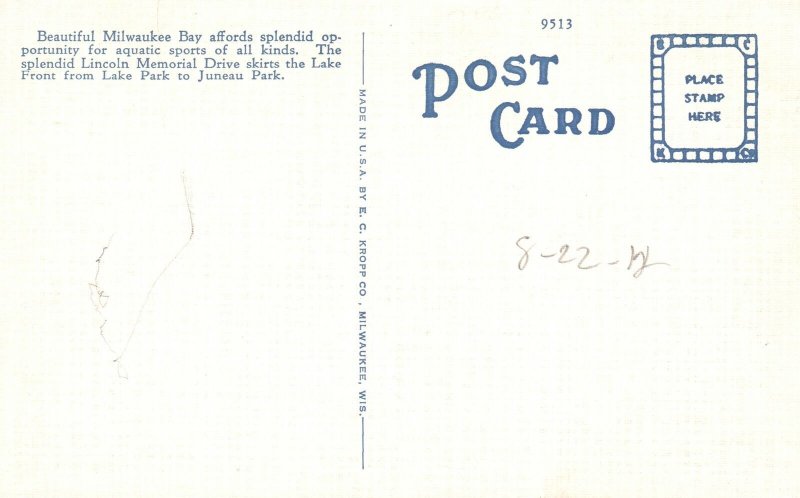This image shows the back of an old, off-white postcard, probably from the 1950s or 60s. The postcard is divided into two halves by a vertical line down the center, with the words "Made in USA by C. Crowe Company, Milwaukee, Wisconsin" written along the line. On the left side, in blue text, it reads, "Beautiful Milwaukee Bay affords splendid opportunity for aquatic sports of all kinds. The splendid Lincoln Memorial Drive skirts the lakefront from Lake Park to Juneau Park." The right side features the larger word "Postcard" in black lettering, with small numbers "9513" above it. There is a rectangle in the top right corner, bordered by squares, with the text "Place Stamp Here" indicating where to affix a stamp. Additionally, at the top, there appears to be a handwritten date that begins with "8-22-" and possibly "12" following it. The space below this is intended for writing the recipient's address, and it remains mostly blank. The overall design and details like the pen or pencil markings suggest the postcard is quite vintage.